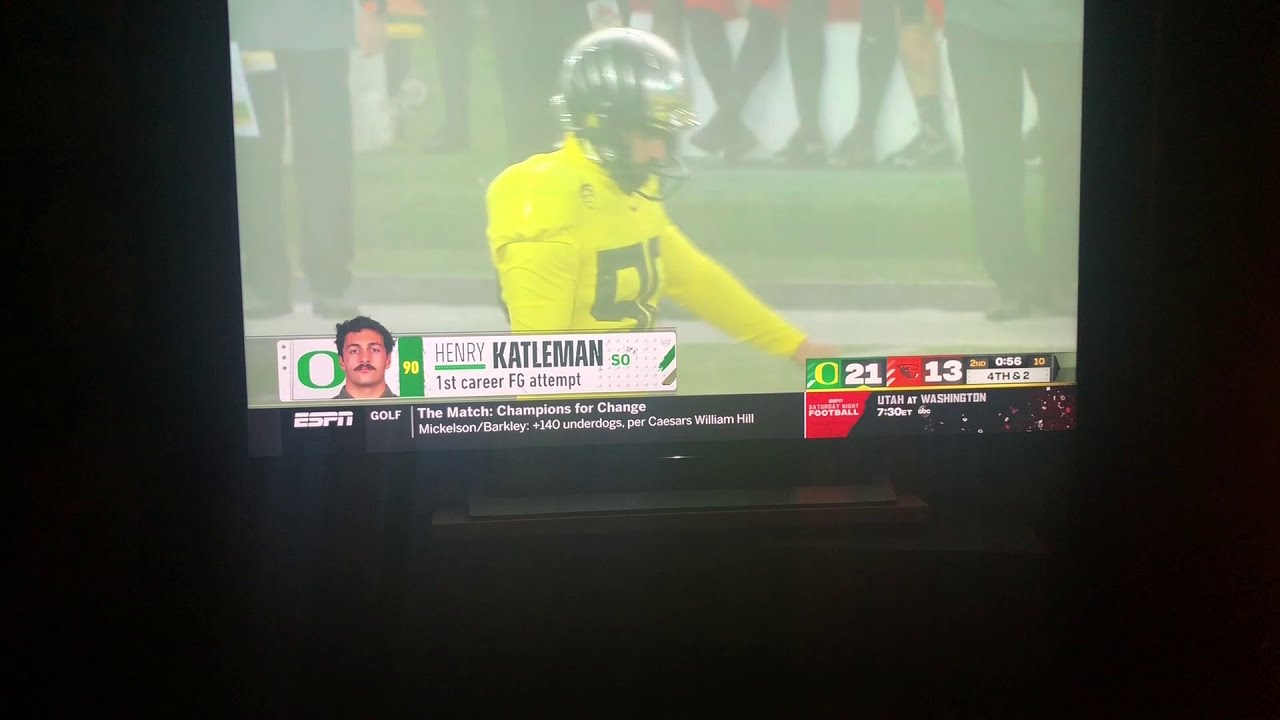The image is of a television screen displaying a college football game featuring the Oregon Ducks against Oregon State. The screen is somewhat hazy, but the key details are visible. Central to the image is Henry Cattleman, the field goal kicker for Oregon, identified by his yellow jersey and silver helmet, bearing the number 90. The text overlay indicates it is his first career field goal attempt. On the bottom right of the screen, the score reads Oregon 21, Oregon State 13, with 56 seconds remaining in the second quarter, and the down and distance is 4th and 2. Additionally, at the bottom of the screen, there is an ESPN logo along with an update on a golf match stating "The Match: Champions for Change" with Mickelson and Barkley as +140 underdogs per Caesars William Hill. The edges of the screen appear dark, possibly due to shadows, and the sidelines are visible, with people watching the game.